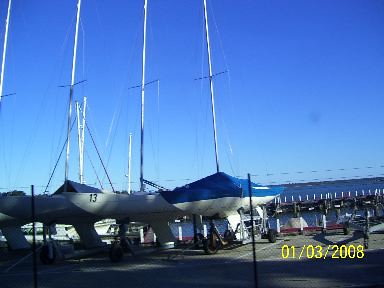The image, dated 01-03-2008, captures a harbor scene under a clear, vibrant blue sky with no clouds in sight. Three small sailboats are prominently featured, docked on land rather than water. The boats are positioned from the center towards the left side of the frame, with an open space on the right. One sailboat has a dark, rich blue stripe near the top section, while the others are plain white. The boats are stored on wheeled trailers, supported by long, thin structures, and their sails are stowed away. One boat bears the number 13 and another has a blue cover over its main body. In the backdrop, a body of water, likely a lake, contrasts with the lighter sky, along with a visible pier or dock. The bottom right corner of the photograph displays the grainy yellow date stamp, 01-03-2008.